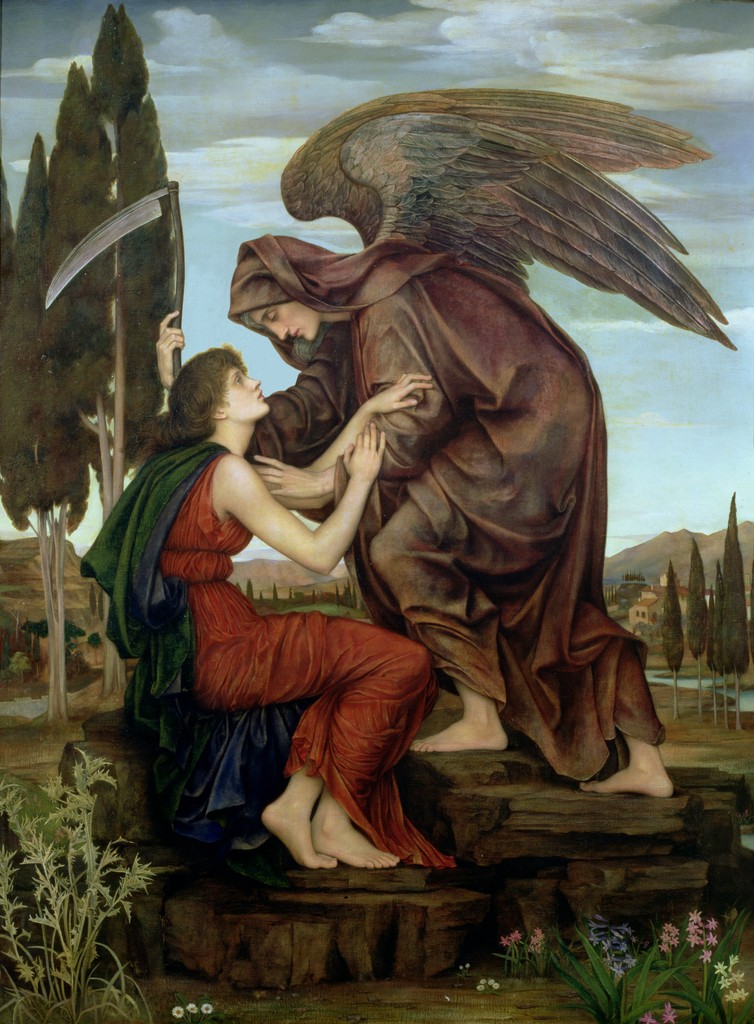This painting, titled "The Angel of Death," portrays a deeply evocative religious scene set in a serene countryside. At the center, a frail woman with short brown hair is wrapped in a rust-colored robe with a green cape. She sits barefoot on a stone bench, gazing up with a look of solemn reverence at an angelic figure beside her. The angel, with androgynous features, is draped in a brown robe and hood, possessing majestic wings with shades of gray and green. In one hand, the angel holds a scythe, reinforcing their somber role, while the other hand rests gently on the woman's shoulder. 

The background is a tranquil blend of tall, thin trees and a distant, mountainous landscape under a clear blue sky, creating a peaceful juxtaposition to the intense focal scene. In the foreground, colorful flowers—blue, pink, and yellow—along with some leafy green weeds, add a touch of life and vibrancy to the composition. This detailed and poignant painting captures the solemn moment of an encounter with the Angel of Death, bathed in both the beauty and the solemnity of its symbolic surroundings.